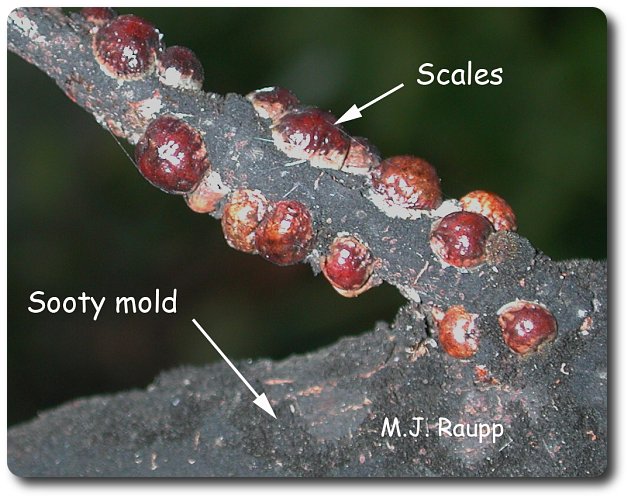This educational close-up image depicts a tree branch afflicted with a black, crusty substance labeled as "sooty mold." The branch, running diagonally from the bottom left to the top right, stands out against a solid green background. Detailed annotations include white arrows pointing to various features; one arrow identifies the sooty mold covering the branch, while another highlights red growths labeled as "scales." The photograph is credited to M.J. Raupp, whose name appears as a watermark in the bottom right corner. This well-labeled and sharply focused image is reminiscent of illustrations found in scientific textbooks, offering an intricate view of the mold and scales present on the branch.